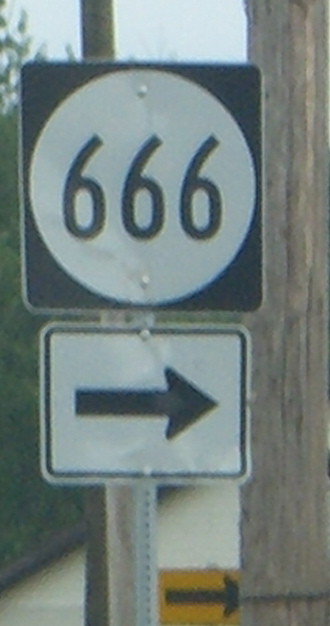The photograph captures a street sign mounted on a silver T-post. The main sign features a white circle with the number "666" in black, enclosed within a black square border, indicating Highway 666. Directly beneath it, a white rectangular sign with a black arrow points to the right. At the very bottom of the image, there's a yellow rectangular sign with another black right-pointing arrow. In the background, partially hidden by trees and slightly blurred, are two wooden power line poles and a glimpse of a building. The sky is visible at the top, forming a subtle backdrop for the scene.